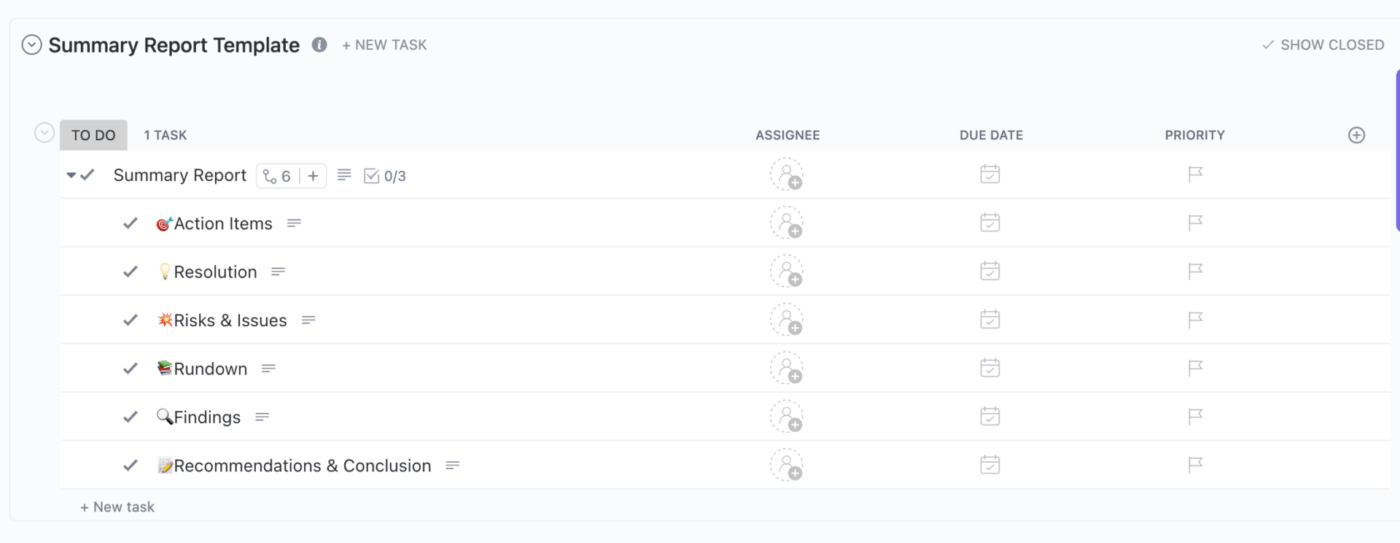The image displays a summary report template featuring multiple sections such as Summary Report, Absentee, Due Date, and Priority, none of which are marked. Additional sections include Action Items, Resolution, Risks and Issues, Rundown, Findings and Recommendations, and Conclusion, all listed under the Summary Report with "To Do" indicators. The purpose of the summary report isn't clear, but the top right corner indicates that the show is closed. Neither the absentees, due dates, nor priorities are highlighted. In the bottom left corner, there's an option to create a new task, suggesting the potential to expand the report over time. The template currently shows one task pending, encompassing all the unmarked items previously listed.